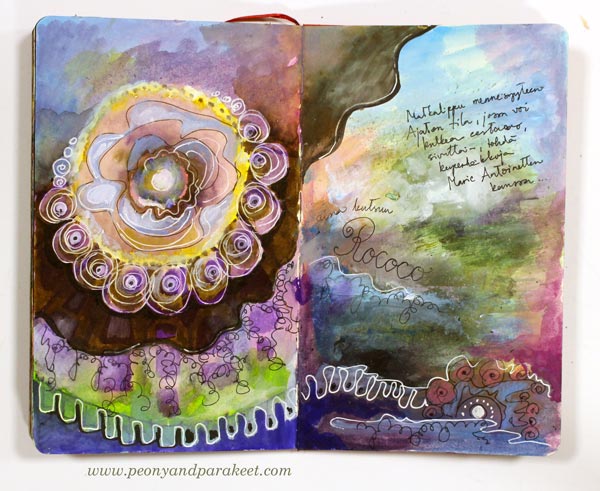The image depicts an open art journal in landscape orientation with a red bookmark hanging out from the top. Both pages are covered in vibrant, abstract watercolor paintings. The left page showcases a circular pattern at the top surrounded by swirling lines in dark green, brown, light purple, and white, transitioning into squiggles and a blend of browns, purples, yellows, greens, and blues at the bottom. The right page features a continuation of the colorful abstract design, intertwined with peach, gray, yellow, and brownish hues. There's a darker green area below fading into blue, with indistinct handwritten text in black ink that appears to include the words "Rococo" and "Marie Antoinette." At the bottom left corner of this page, the website URL www.peonyandparakeet.com is visible. The artwork combines elements of watercolor and marker, merging into a cohesive, multicolored abstract design.